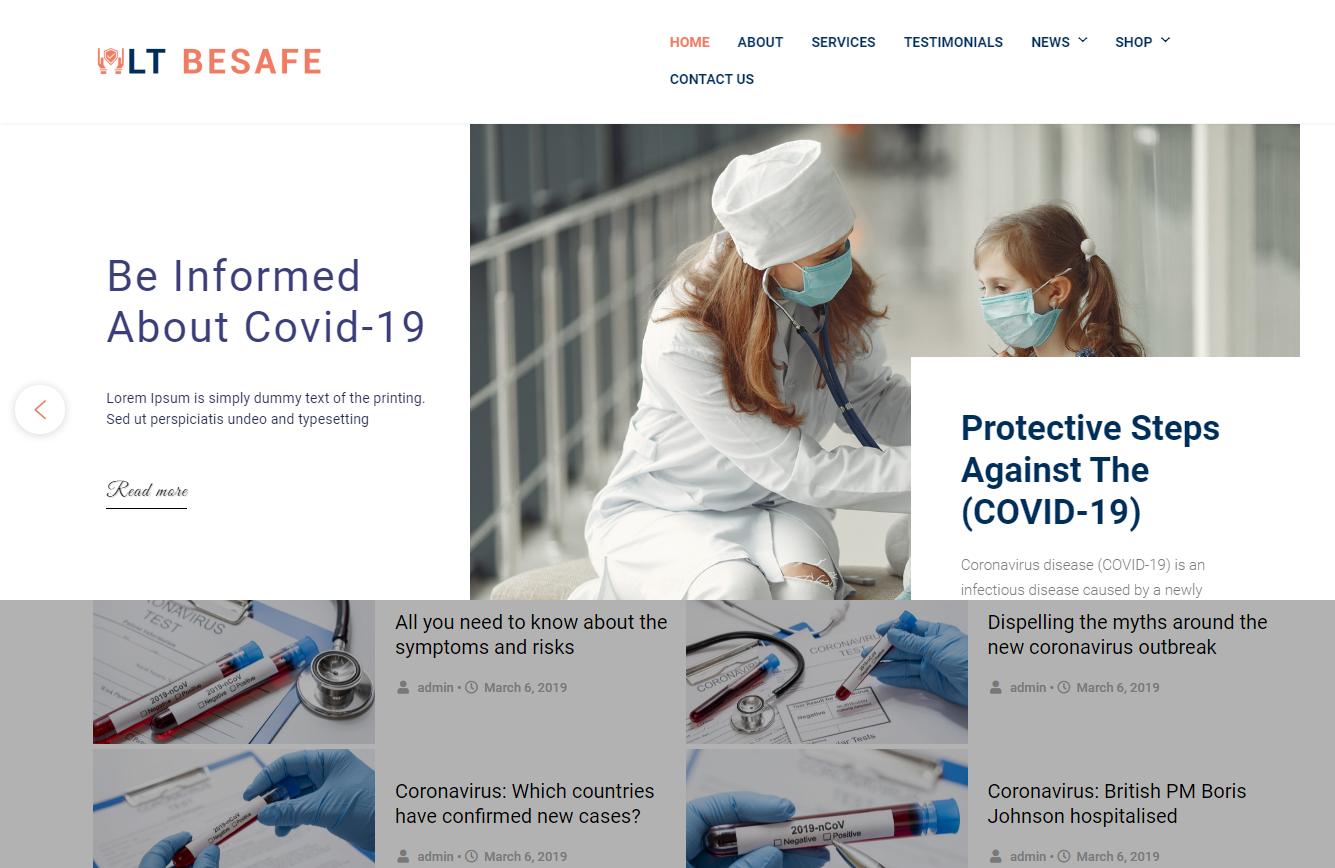This image depicts a medical-themed website with a clean, white background complemented by navy blue and occasional colored text. In the upper left corner, there's an icon featuring two hands and the letters "LT," followed by the phrase "be safe," indicating the website's name, "LTV Safe."

In the top-right corner, the navigation menu includes options such as Home (highlighted in pink), About, Services, Testimonials, News, Shop, and Contact Us.

Prominently displayed on the page is a section titled "Be informed about COVID-19," featuring placeholder text resembling lorem ipsum. Adjacent to this section is a "Read More" link in cursive script.

To the side, there's an image of a female doctor assisting a young girl. Both are wearing protective masks, and the doctor, dressed in white, is placing a stethoscope on the child's chest. This image is accompanied by text that reads, "Protective steps against COVID-19," followed by a truncated description starting with "Coronavirus seen COVID-19 is an infectious disease caused by a newly..."

Below this, several other sections provide information on topics such as symptoms and risks of COVID-19, countries with confirmed cases, myths surrounding the coronavirus outbreak, and a news headline about British PM Boris Johnson being hospitalized due to the virus.